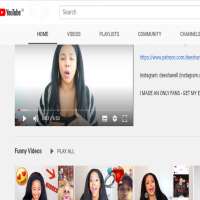The screenshot captures a webpage showcasing a video streaming platform. Prominent sections of the site include navigation tabs for "YouTube Home," "Videos," "Playlists," "Community," and "Channels," though the last tab is partially cut off. 

At the forefront, an African American woman with long black hair and hoop earrings is featured in a video. The video appears to have just started, with a red progress bar indicating that approximately 2% of the content has been played. 

To the right of the video, there are three related links or sections, with one highlighted in blue. 

Below the main video, there is a section titled "Funny Videos," where a "Play All" option is available. This section includes three thumbnails, and the first one shows the same woman smiling with a heart emoji in the background. 

Overall, the layout suggests an organized platform emphasizing easy navigation and related content discovery.